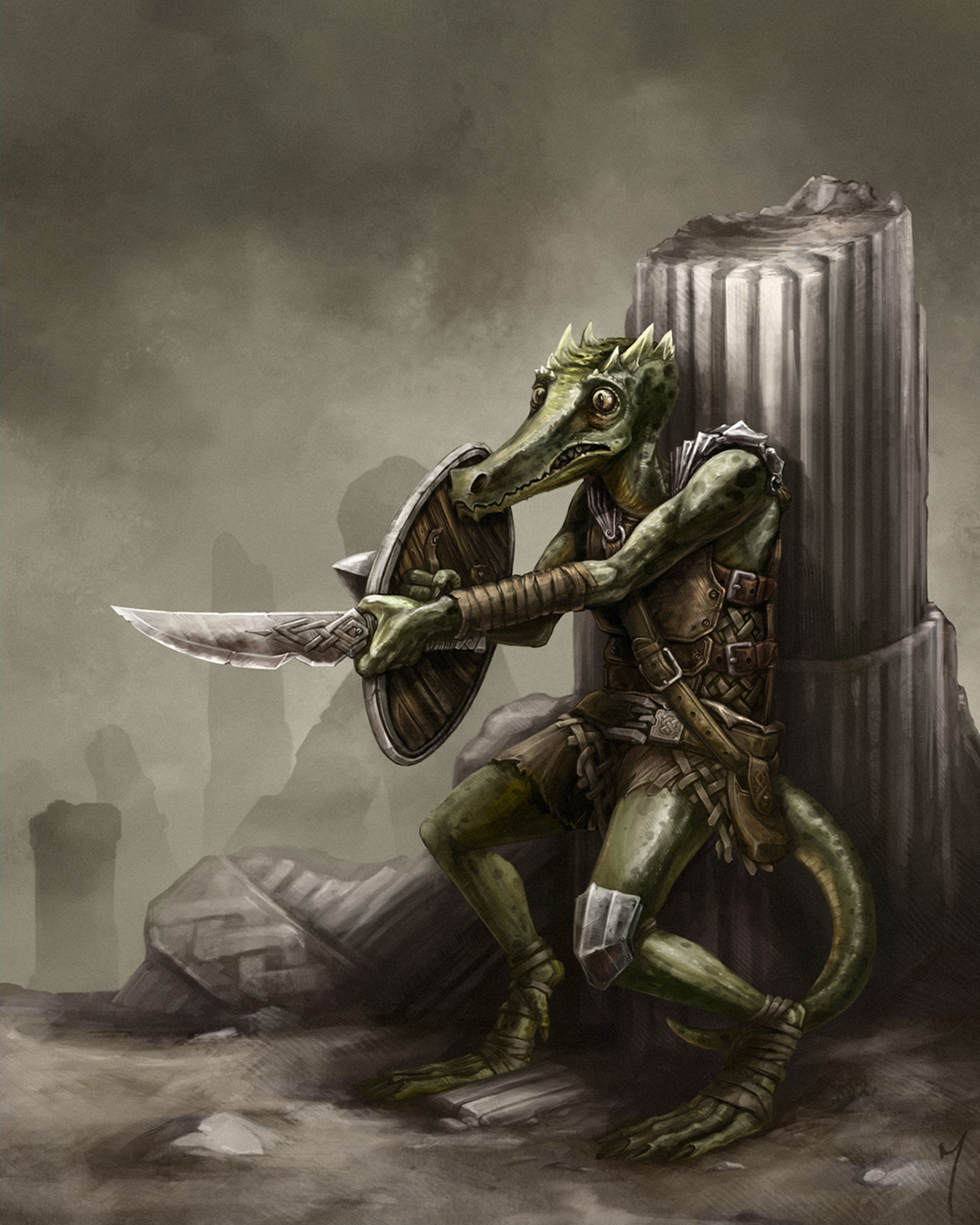In this detailed digital illustration, a dragon-like creature, reminiscent of an alligator with green scales, stands amidst a gray, smoky, and misty battlefield. The background is dotted with multiple broken columns, rendered in black and white, casting an eerie, shadowy atmosphere. The main focus is a partially destroyed column behind the creature, against which it is backed up, suggesting a scene of recent turmoil.

The creature is adorned in worn, brownish armor, which includes a steel knee plate on its left knee and additional protective gear on its chest. Its large, wrapped feet clutch the ground, while its forearms are similarly wrapped, hinting at a readiness for combat despite its apparent fear. The nervousness is palpable in its exceedingly large eyes and its overall posture. 

The beast clutches a knife with intricate Celtic markings and points it directly in front, towards the left side of the scene, signifying its defensive stance. In its other hand, it holds a shield, providing extra protection. The creature's head is crowned with a series of white horns, adding to its mythical appearance, while its long tail trails behind it, completing the image of a beleaguered yet resilient warrior in a desolate and hauntingly vivid scene.